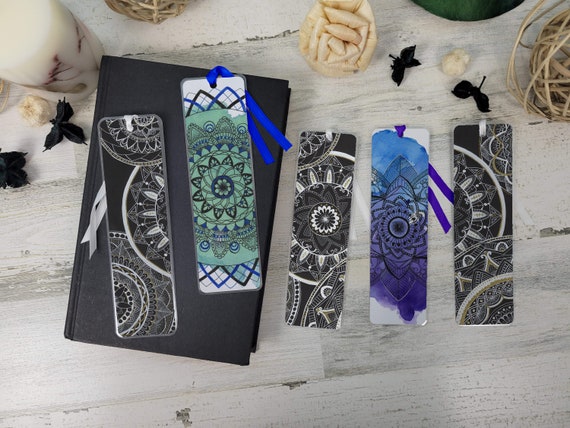This top-down photograph captures a meticulously arranged scene featuring five distinct bookmarks, each adorned with intricate designs reminiscent of spirograph and sacred geometry patterns. These bookmarks, possibly made of plastic, display a variety of color schemes: three in stark black and white, and two more vibrant ones in shades of purple and green. The bookmarks showcase unique, cropped circular designs, with patterns outlined in contrasting colors. Each bookmark is adorned with a tassel through a hole at the top, colored white, blue, or purple. They are elegantly laid out on a grayish wood table, which also holds a black book on the left and various decorative items, such as candles, a wooden ball, and feathers, enhancing the aesthetic appeal.